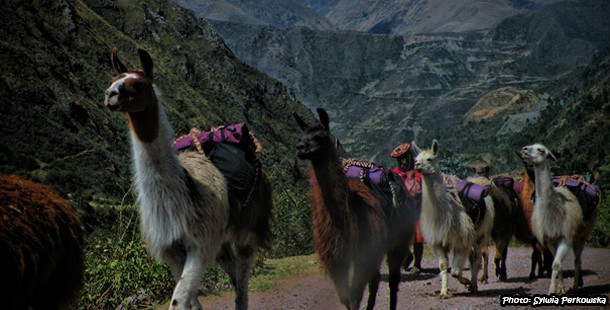The image depicts a picturesque, mountainous landscape in a remote hilly location during daylight. A herd of llamas, adorned with purple cloths and black packs, are ascending a dirt road that winds up the mountainside. The llamas, with their brown, white, and mixed-colored fur, appear alert and determined as they march from right to left. Accompanying them is a person with dark brown skin, dressed in traditional attire featuring a red hat and tunic, walking slightly behind the animals. The backdrop consists of rugged grey and green mountains, some featuring rocky outcrops and others dotted with grasses and trees. The scene captures the essence of a journey through a breathtaking yet demanding terrain. In the bottom right corner of the photo, a watermark credits the image to Sylvia Perkovska.